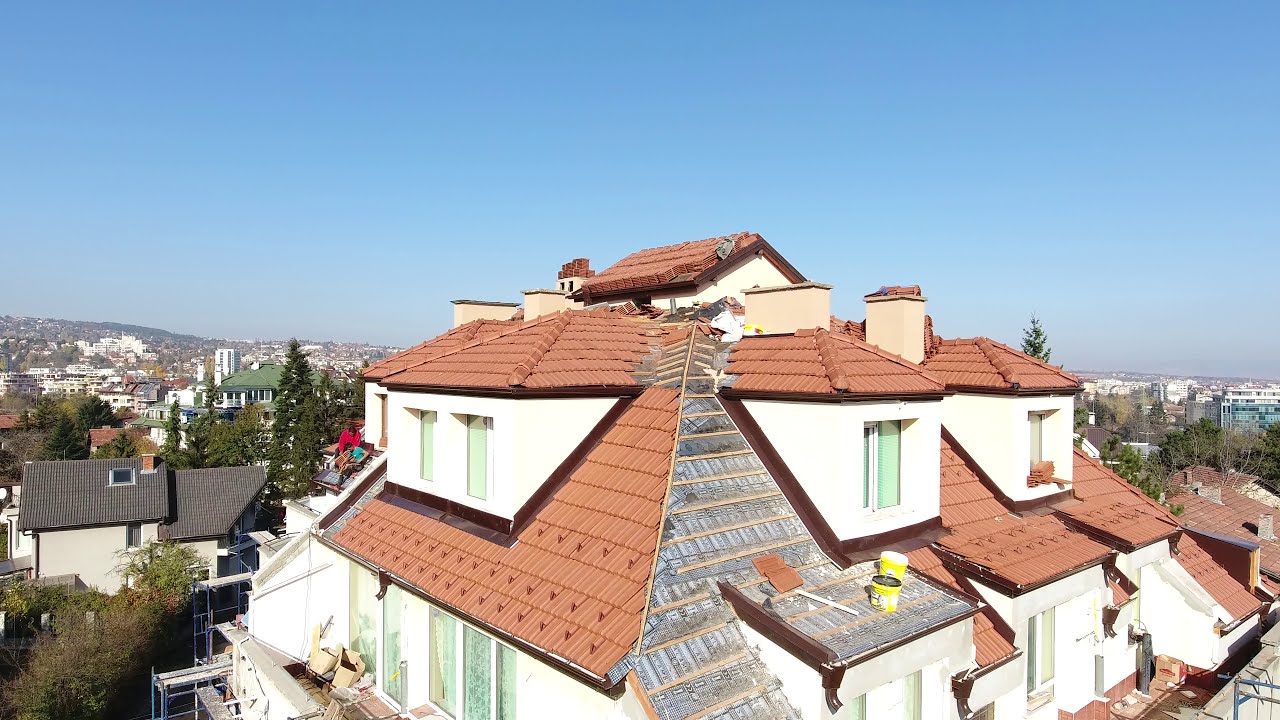This horizontally aligned rectangular image presents a clear, cloudless blue sky that progressively deepens in hue from light to dark as it rises, occupying the top half of the picture. The vantage point, taken from a height roughly level with the third story of a building, showcases the ornate architecture of a large house with intricate design elements. The house, characterized by its reddish-brown or maroon clay roof tiles, has a unique structure featuring sloping roofs and multiple dormer windows. The bright stucco-like white walls accentuate the numerous stone-framed windows that punctuate each side of the building, and cream-colored chimney stacks rise from the roof.

One prominent section of the roof, positioned centrally in the image, is under construction, evidenced by tall yellow and white buckets and a lack of shingles. Surrounding this main structure, the landscape extends into the distance on both the left and right sides, revealing more buildings, possibly apartments, with similar architectural styles and varied roof colors. Trees with green foliage interspersed among the buildings add a natural element to the scene. In the left background, closer to the frame, another house with a brown roof and white stone walls is visible. Far off on the horizon, a multitude of white buildings can be seen, blending distinctly with the serene blue sky above.